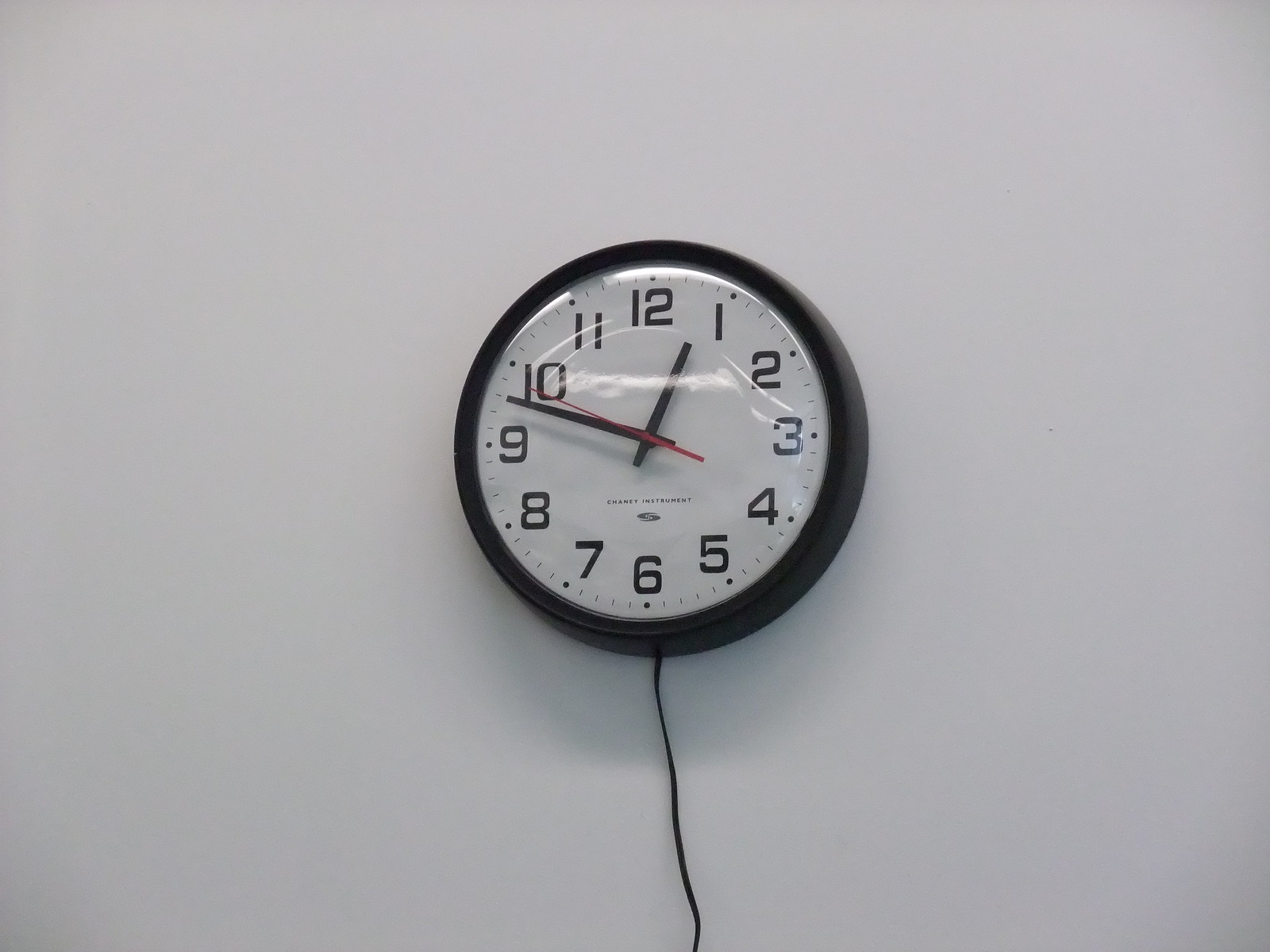This image features a standard office wall clock with a glass case cover. The clock face is white, displaying black numbers marked by small dots at each numeral. Thin black lines segment the spaces between the numbers, and the clock's hands are also black, while the second hand stands out in red. Near the 11 o'clock position, there appears to be a chip or some form of distortion on the glass, impacting the clarity of the clock face. Additionally, the glass surface reflects ambient light from above. A black wire, likely for power, runs down the gray wall starting at the six o'clock position. The wall itself is a light gray color, contributing to the typical office decor.